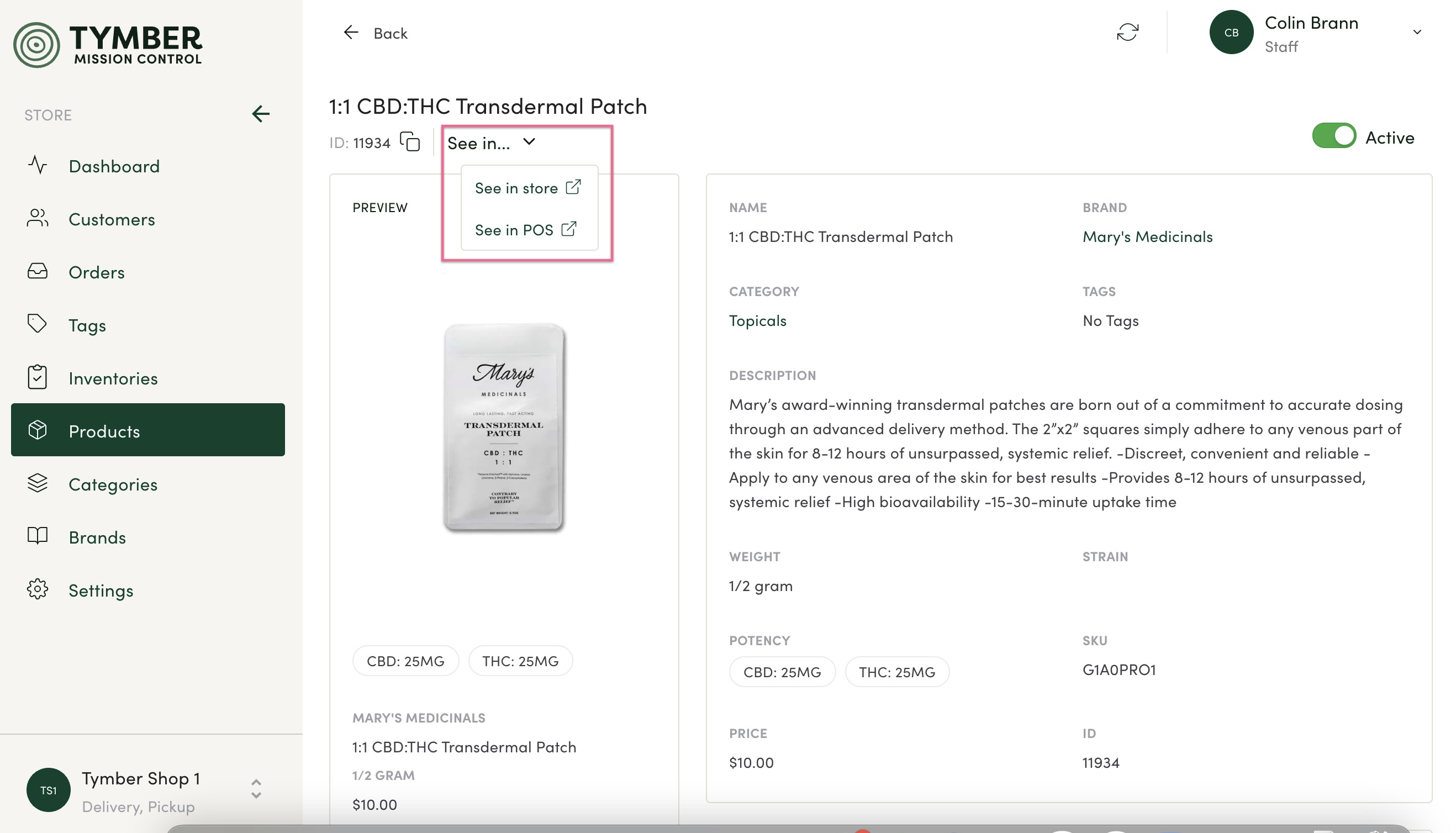The screen displays the user interface of Timber Mission Control, highlighting various navigation options and detailed information for a specific product. At the top of the interface, labels such as "Store," "Dashboard," "Customers," "Orders," and others are visible, with "Products" currently highlighted. Towards the center, "Timber Shop 1" is indicated with an up and down arrow next to it, along with options for "Delivery" or "Pickup."

On the top right corner, there's a green "Active" button switched on. Under this section, detailed information about a product is presented:

- Product Name: CBD+THC Transdermal Patch
- Type: CN (Cannabinoids)
- Purchase Options: Available via a dropdown menu labeled as "See in Store" or "See in PLS"
- Image: Displays the patch itself
- Specifications: 
  - Weight: 0.5 grams
  - Price: $10
  - Brand: Merry Medicinals
  - Category: Topicals
  - Tag: No Tags
  - Strain: Blank
  - Potency: 25 mg CBD + 25 mg THC
  - Product ID: 11934

This allows users to see comprehensive product details, including price, potency, and additional categorization information, all within the streamlined interface of Timber Mission Control.